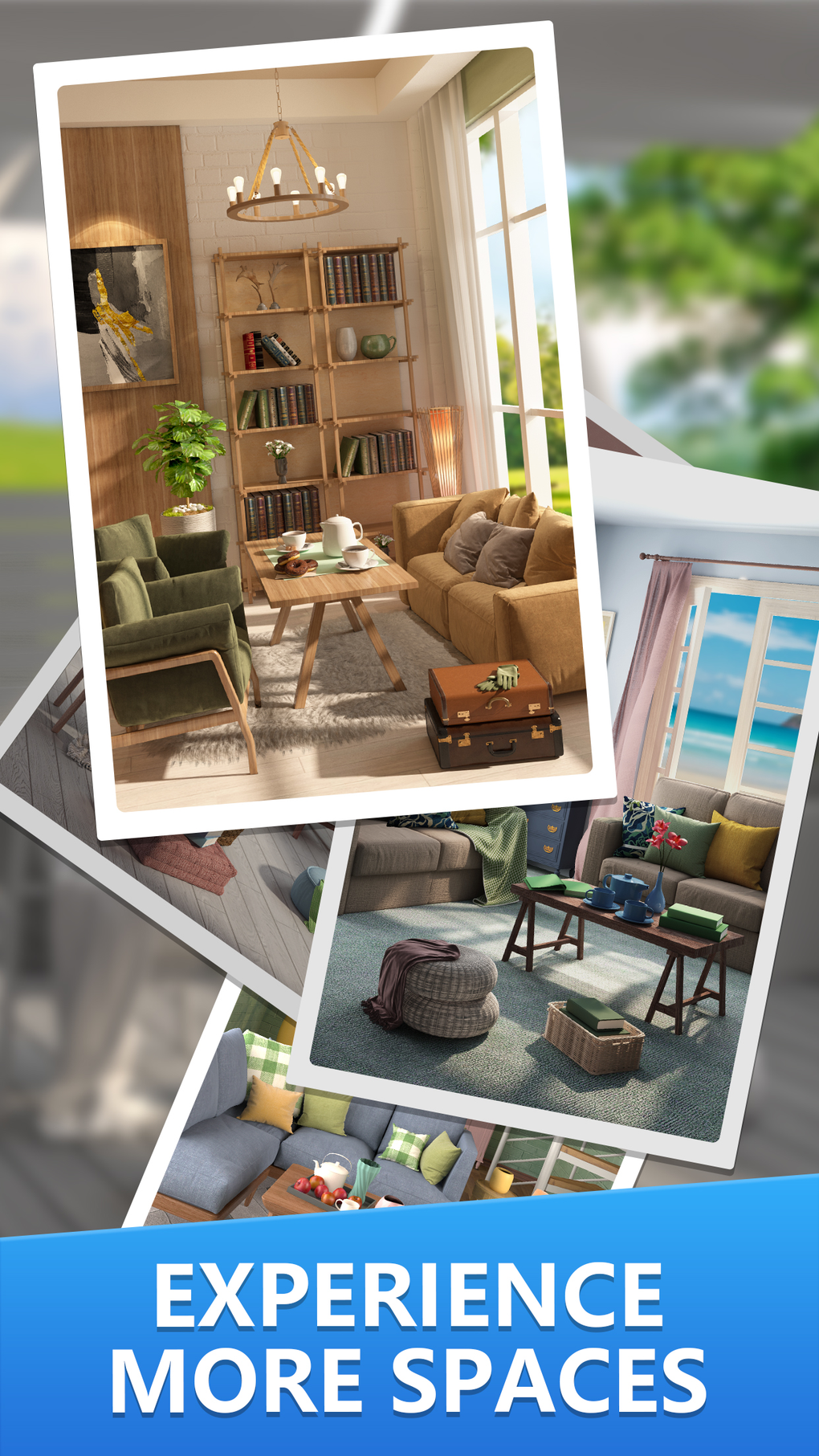This screenshot appears to be from an advertisement or a website showcasing interior design renderings. The layout consists of four floating, white-bordered images that resemble casually arranged, high-quality snapshots of home interiors. These images are set against a blurred background scene featuring trees visible through a window, adding to the overall depth and dimension.

1. **Top Image**: Displays a cozy home interior with a well-stocked bookshelf, a lush green plant, comfortable sofas and chairs, suitcases on the floor, and a chandelier. A coffee table adorned with donuts and tea completes this inviting setting.
2. **Second Image (Top Right)**: Positioned at an angle, it presents a room with a fake seascape visible through a window, indicating the use of digital rendering rather than actual photographs.
3. **Third Image**: Features a stylish pouf draped with a throw, accompanied by a sleek coffee table - typical elements of modern interior design.
4. **Fourth Image**: Similar in style to the previous ones, showcasing more elements of contemporary home interiors.

At the bottom of the screenshot, bold white capital letters with a blue drop shadow state "EXPERIENCE MORE SPACES." This text is placed against a blue background, which angles upward from left to right at about a five-degree incline, creating a dynamic visual effect.